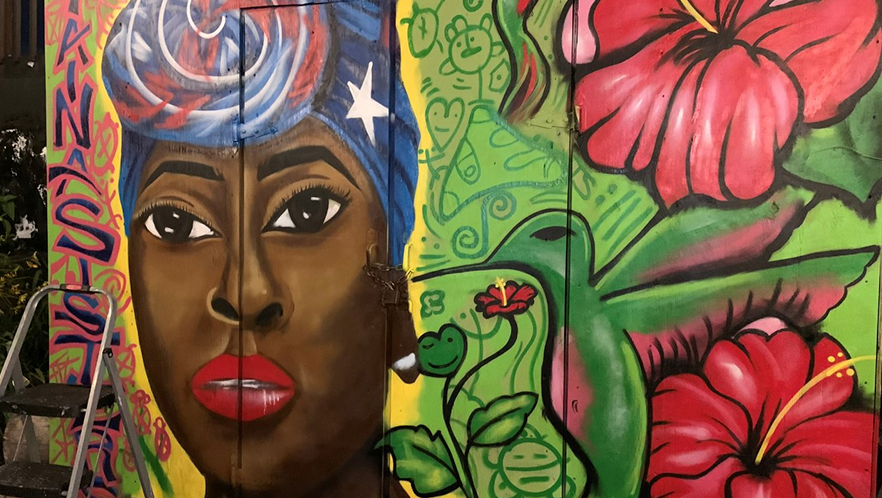The mural, painted in an artistic graffiti style, features a detailed and colorful depiction of an African woman on the left-hand side. She has brown eyes, which are open, and black trimmed eyebrows accentuating her face. Her bright red lips, enhanced with lipstick, are slightly parted, revealing her teeth. The woman wears a vibrant cloth head wrap adorned with a white star, predominantly blue with red accents, and a gold nose ring on her right nostril. Surrounding her, to the right side of the mural, are pink and red flowers, likely roses, interspersed with green leaves and plants. A green hummingbird is positioned next to her face, adding to the natural elements of the mural. The entire artwork is bolstered by the rich palette that includes pink, dark pink, yellow, dark green, red, blue, white, black, brown, and gold colors. Text adorns the left-hand side of the mural, though it is not fully legible. A step stool is propped against the wall in front of the mural, suggesting its use by the artist to reach higher sections while painting.